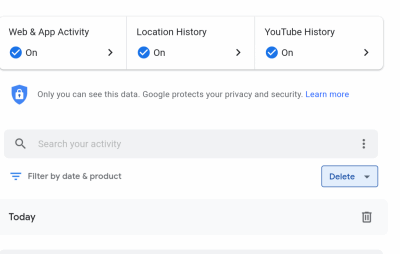A screenshot displays a web dashboard with a clean white background. The interface prominently features the section titled "Web & App Activity," accompanied by blue checkmarks indicating that "Location History" and "YouTube History" are enabled. The dashboard allows users to filter activities by date and product and includes a "Delete" button alongside a trashcan icon for easy removal of entries. A search bar with the placeholder text "Search your activity" is also visible, inviting users to search through their stored activities. The overall design is minimalist, providing a clutter-free user experience. Though the exact purpose of the dashboard is ambiguous, it appears to be part of a web interface template or an activity monitoring tool.